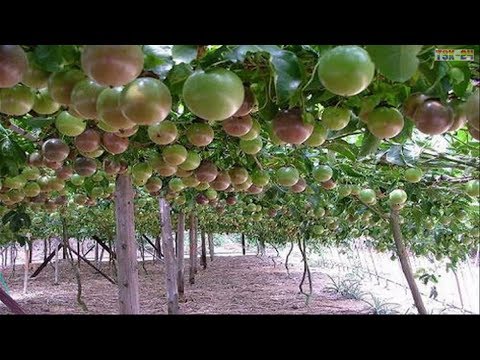This image features a vast orchard or plantation where rows of trellis-supported apple trees stretch into the distance, creating a dense canopy of green. The primary focus is on the multitude of apples hanging from the branches, in various stages of ripening. The apples exhibit a range of colors, from green to reddish-green to deeper reds, indicating their ripening process. The orchard floor is predominantly bare, characterized by brown soil with sparse leaves, giving it a clean appearance. In the foreground and mid-ground, the profuse leaves and vines create a verdant backdrop, accentuating the vividly colored apples. Beyond the orchard, patches of tall green grass are visible, marking the edges of this meticulously maintained grove. The image, bordered by wide black bars on the top and bottom, provides a panoramic view that immerses the viewer in the tranquil yet lush setting of the apple orchard.